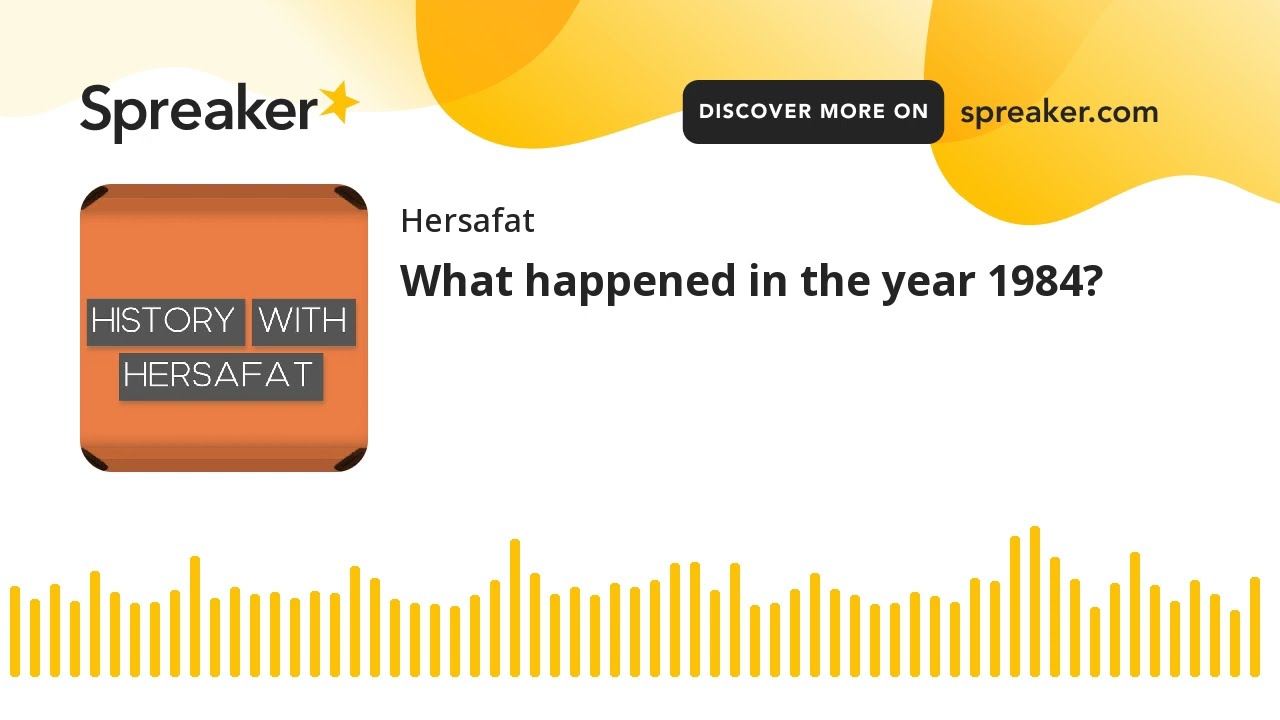The image is a wide rectangular digital ad with a predominantly white background, featuring various graphic elements and text. In the upper left corner, the word "Spreaker" is written in black font next to a gold five-pointed star. On the upper right, within a black rectangle with curved corners, the text in white font reads "Discover More On," followed by "Spreaker.com" in black letters.

Central to the image, there's an orange square with rounded corners that overlays a gray rectangle, containing the white text "History with Hersefat." To its right, the bold black letters declare, "Hersefat: What Happened in the Year 1984." The top quarter of the image is adorned with yellowish-orange patterns, featuring curved lines and shapes of differing intensities and paleness, adding a dynamic aesthetic.

The bottom of the ad showcases a series of vertical, uneven yellow rectangles, suggestive of audio waveforms, reinforcing the idea that the content is likely related to an audio podcast. Overall, the design is modern with recurring thematic colors of yellow and orange, accentuated by black and white text elements to highlight critical information about a podcast titled "History with Hersefat."